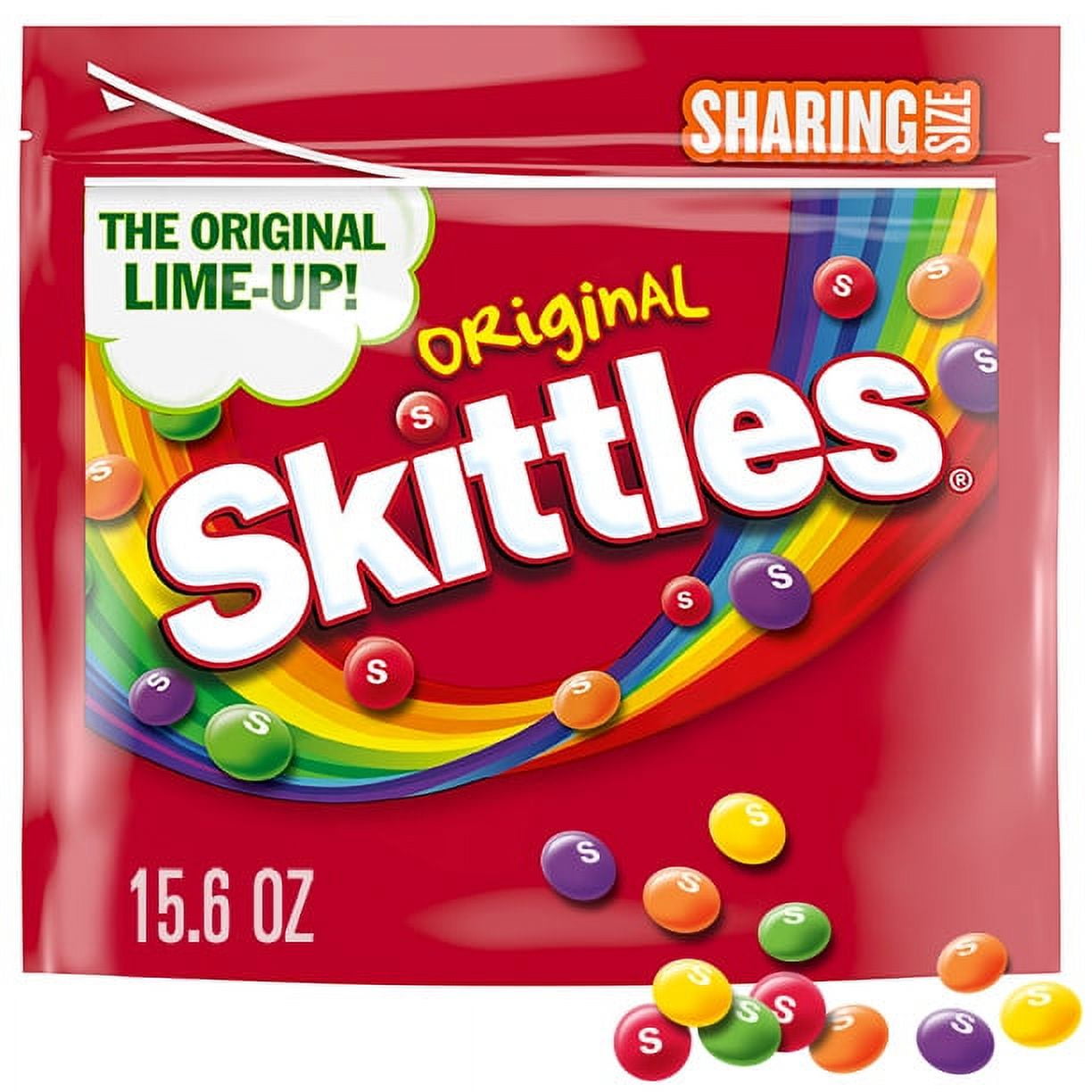This is an advertisement illustration for Skittles featuring a large red bag labeled "Sharing Size" in white text with an orange border on the top right corner. The packaging prominently displays "The Original Line-Up" and "Original Skittles," with the latter written in big white font with a red border and a trademark "R" symbol. A rainbow, designed to resemble a smile, arches across the bag, showcasing Skittles in various colors: red, orange, yellow, green, purple, and possibly others. Below the bag, a playful cascade of colorful Skittles spills into the foreground, creating a vibrant and artful effect. The total weight is specified as 15.6 ounces (OZ) in the bottom left corner. The Skittles are depicted with their iconic white "S" markings reaffirming the lively and enticing nature of this advertisement.